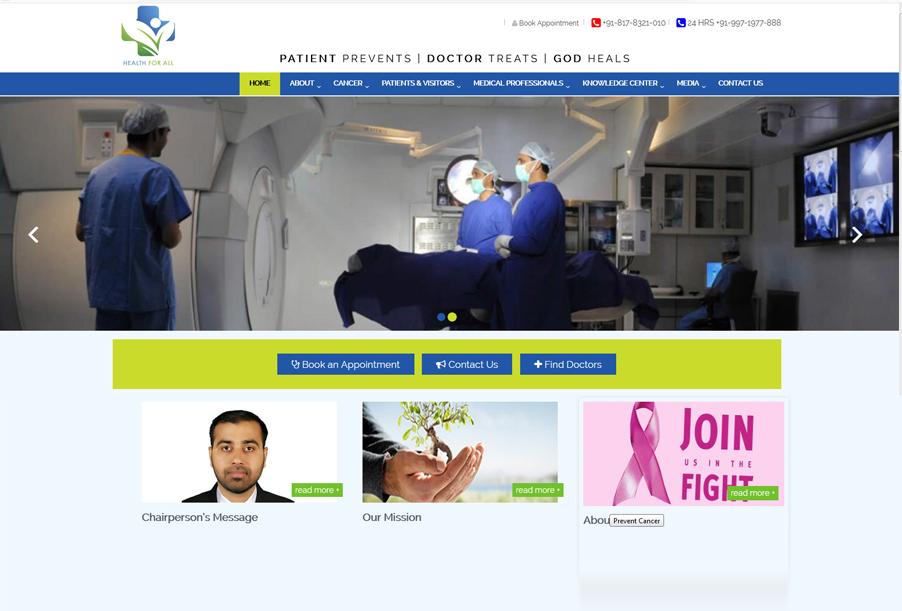The image showcases the homepage of a medical website named "Health for All," prominently displayed in the upper left corner alongside a unique logo that combines a cross with plant elements against a blue background. The top section of the site features a clean white background. On the top right, there are links for booking appointments and two phone numbers: one with a red phone icon, likely representing regular business hours, and another with a blue phone icon signifying 24-hour emergency support.

The top bar is blue and includes an inspiring motto: "Patient Prevents, Doctor Treats, God Heals," hinting at the organization's religious affiliation. The navigation menu provides links to several sections: Home, About Cancer, Patients and Visitors, Medical Professionals, Knowledge Center, Media, and Contact Us.

Centrally positioned is an image depicting several medical professionals in scrubs, seemingly preparing for a procedure. Below this image are three prominent call-to-action buttons: "Book an Appointment," "Contact Us," and "Find Doctors." The bottom section of the homepage displays three advertisements highlighting their chairperson's message, mission statement, and additional information about the organization.